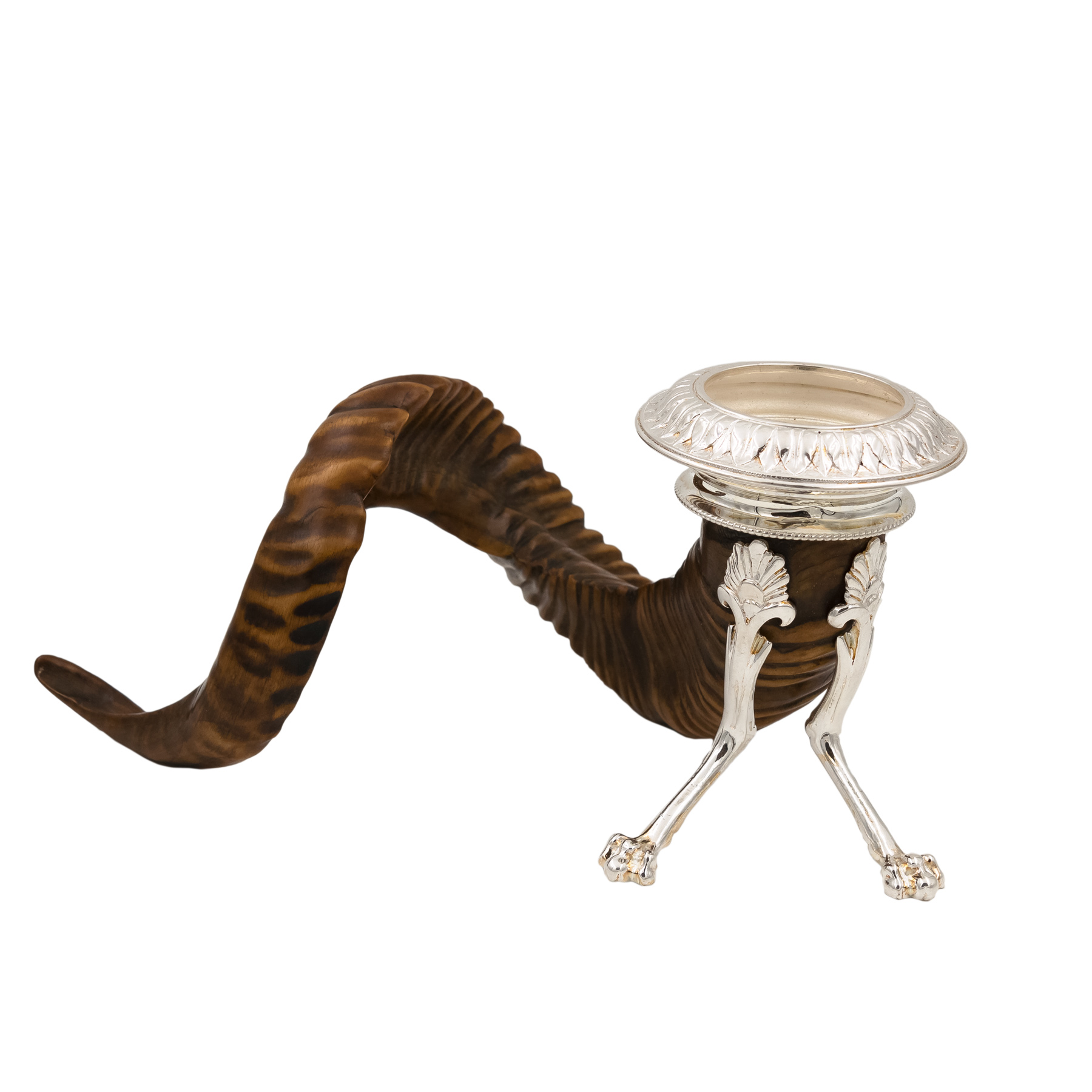This photograph showcases a unique and intriguing ornament, isolated against a clean white background, suggesting a professional presentation possibly intended for an online marketplace. The main body of the object appears to be crafted from dark brown wood with lighter brown patterns, featuring pronounced ridges along its length, giving it a textured, almost bumpy feel reminiscent of a natural ram's horn or possibly even an antique pipe. This horn-like shape curls gracefully, ending with a smooth, shiny metal top, likely stainless steel or sterling silver, fashioned into a decorative, intricately made candle holder. Adding to its ornate charm, the piece includes two silver legs attached to the base, enhancing its collectible and antique-like appearance. This visually striking item, blending natural aesthetics with metal craftsmanship, could potentially serve as a unique decorative piece or a sophisticated collectible.